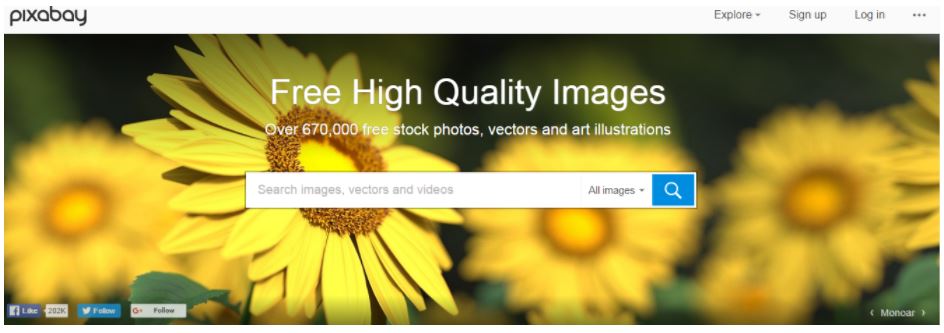The image depicts the homepage of Pixabay, a website known for offering free, high-quality images. At first glance, the website highlights its extensive collection, boasting over 670,000 free stock photos, vectors, and art illustrations available for use in both commercial and personal projects. The user-friendly interface encourages users to search for any type of image they need. The focal point of the homepage features a clear, front-facing layout with subtle background details. The background prominently showcases sunflowers, which are artistically blurred to emphasize one of the many high-quality images accessible through Pixabay without detracting from the main content. The overall design and color scheme of the website exude a creative vibe, reinforcing its utility as a valuable resource for various project needs.